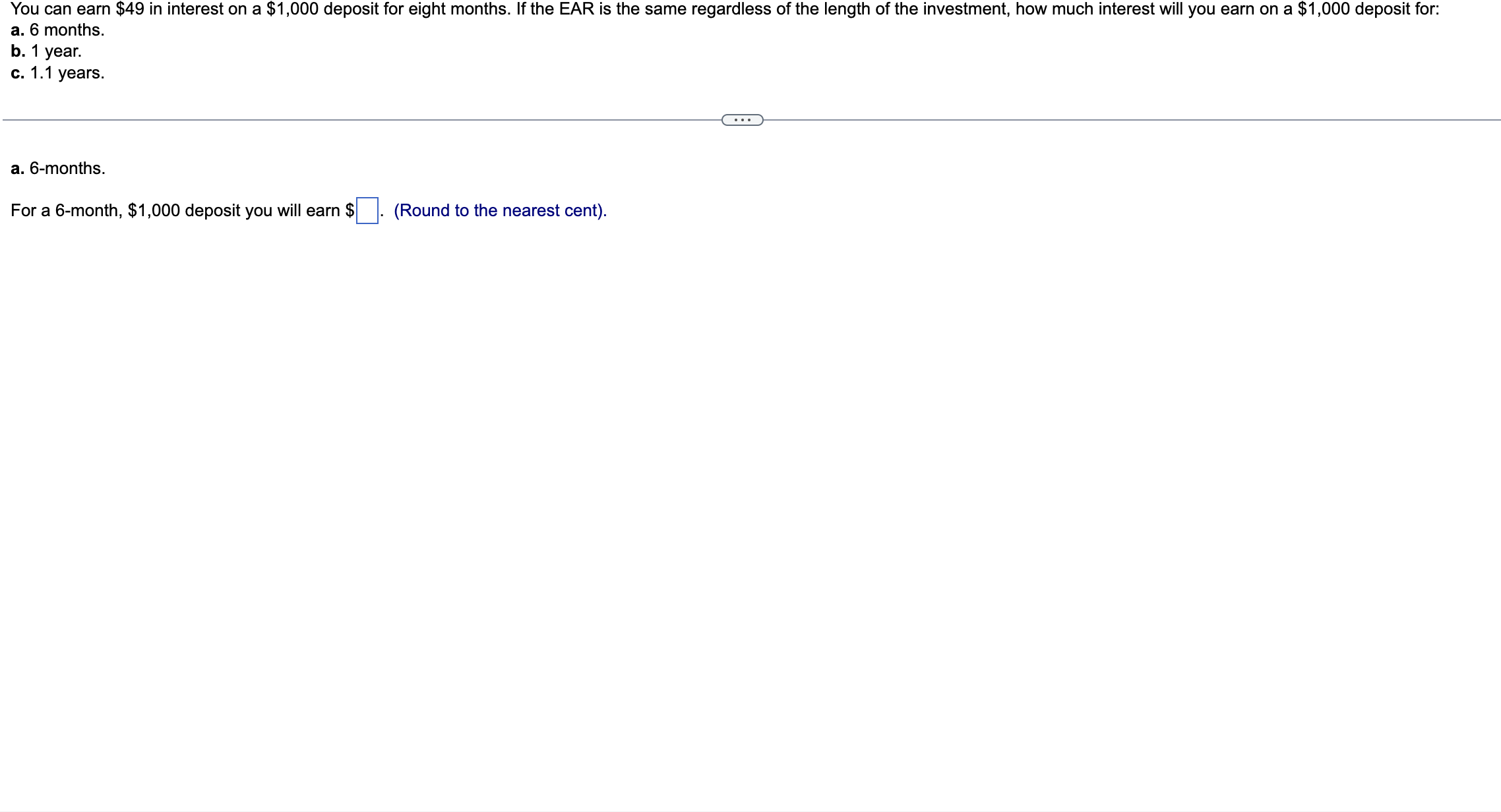This image captures a screenshot of an educational webpage or digital document with text set against a white backdrop. The header at the top reads: "You can earn $49 in interest on a $1000 deposit for 8 months if the annual interest rate is constant regardless of the investment duration. How much interest will you earn on a $1000 deposit for A. 6 months B. 1 year C. 1.1 years?"

Beneath this text, a horizontal gray bar spans the width of the image. At the center of the bar is a small oval containing three dots, effectively separating the top section of the document from the bottom.

In the lower section, the document begins to address the query posed earlier. It starts with "A. 6 months." Directly below this, there is an instruction for calculating the interest earned on a $1000 deposit over a 6-month period. Following this, a blank input box is provided for the user to enter their answer. In blue text to the right of the input box, and enclosed in parentheses, it says "round to the nearest cent."